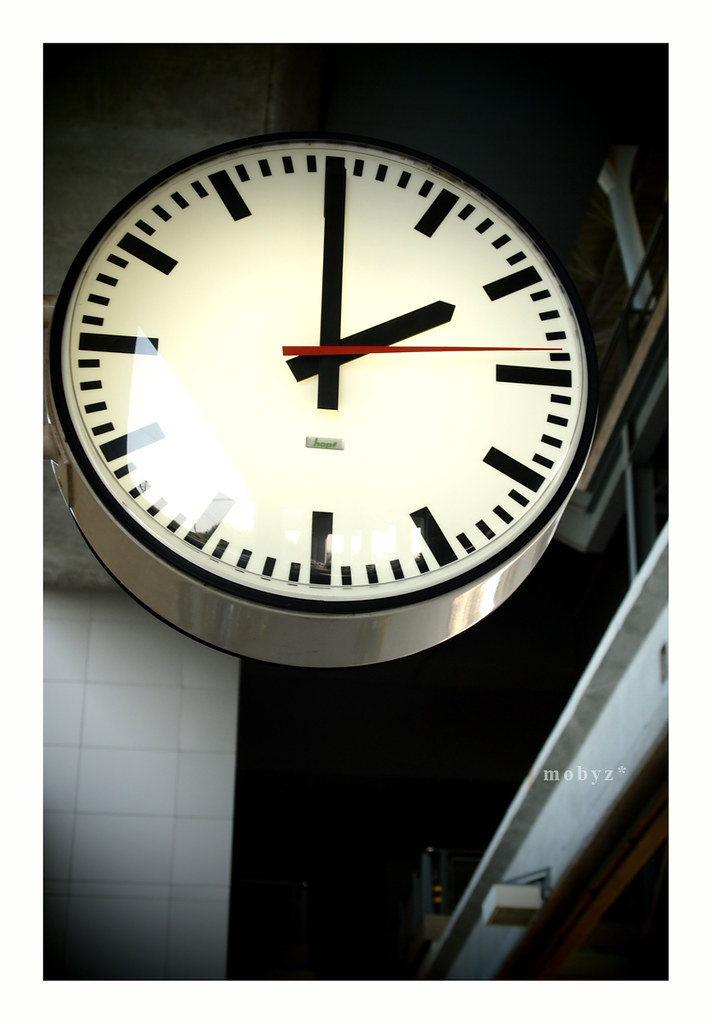This detailed caption describes an image of a traditional school clock:

"A traditional school clock, devoid of any numerical markings, features two hands and a prominent bright red second hand. The clock's face is marked at its corners with black indicators. At its center, a green tag labeled 'Hops' is visibly affixed. In the bottom corner of the clock's face, a label reading 'Moby's' in white letters, accompanied by a small star, suggests it might be attributed to the photographer. The clock is mounted on the side of a wall, set against a background of white brick, with notable black accents. The setting appears to be an open hallway with high ceilings, evocative of a school environment."